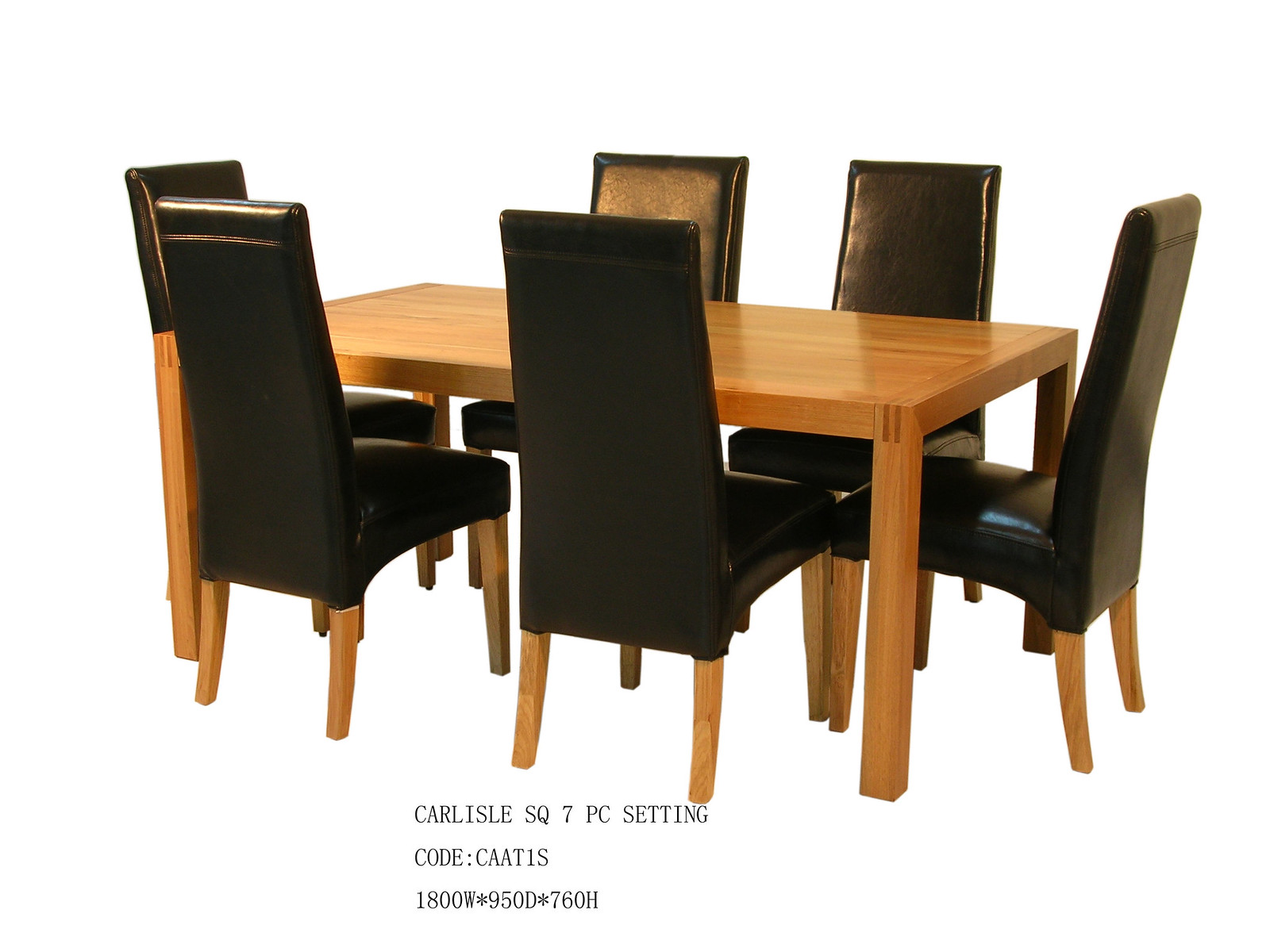This image is a highly detailed, realistic photograph of a dining set on a pure white background, suggesting it was either edited digitally or photographed in a studio. At the center of the composition is a rectangular dining table made of light brown, polished wood with four sturdy legs. Surrounding the table are six high-back chairs, each featuring black, leather-like cushioned surfaces on both the front and back, providing a sleek and smooth aesthetic. These chairs also have legs made of the same light brown wood as the table, creating a cohesive design. The chairs are arranged with one at each end of the table and two along each long side. In the bottom left corner of the image, there is black text that reads: "CARLISLE SQ7 PC setting, code: CAAT1S, 1800W * 950D * 760H," specifying the product details and dimensions. This setup, devoid of any background elements, emphasizes the dining set as a feature likely intended for a retail advertisement.